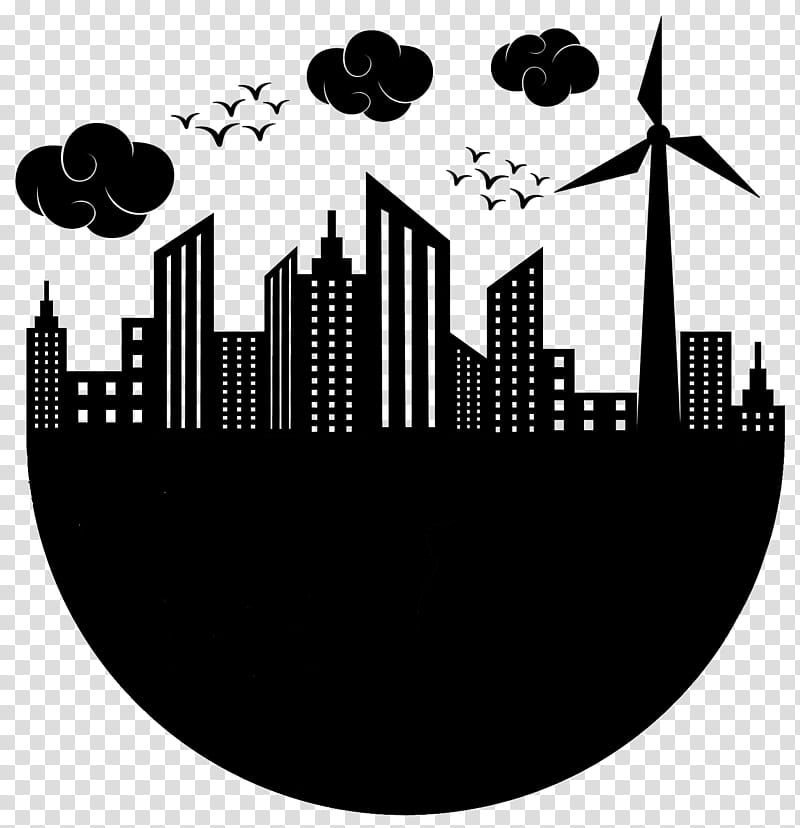This PNG image is a detailed vector illustration of a generic cityscape. The background consists of a grey and white checkered pattern, indicating transparency. The lower half of the image features a solid black semicircle that serves as the base. Rising from this base is an array of skyscrapers and tall buildings, depicted as black silhouettes with white square-like windows. Notably, the middle section contains the tallest buildings, emphasizing the metropolitan feel. To the far right, a smaller structure resembling a church can be spotted. Dominating the right side is a large modern windmill with three blades, its height reaching up into the sky. The sky above the city is populated with three uniquely designed swirling clouds and two flocks of V-shaped birds, all rendered in black to match the minimalist, pencil-drawn style of the city below.